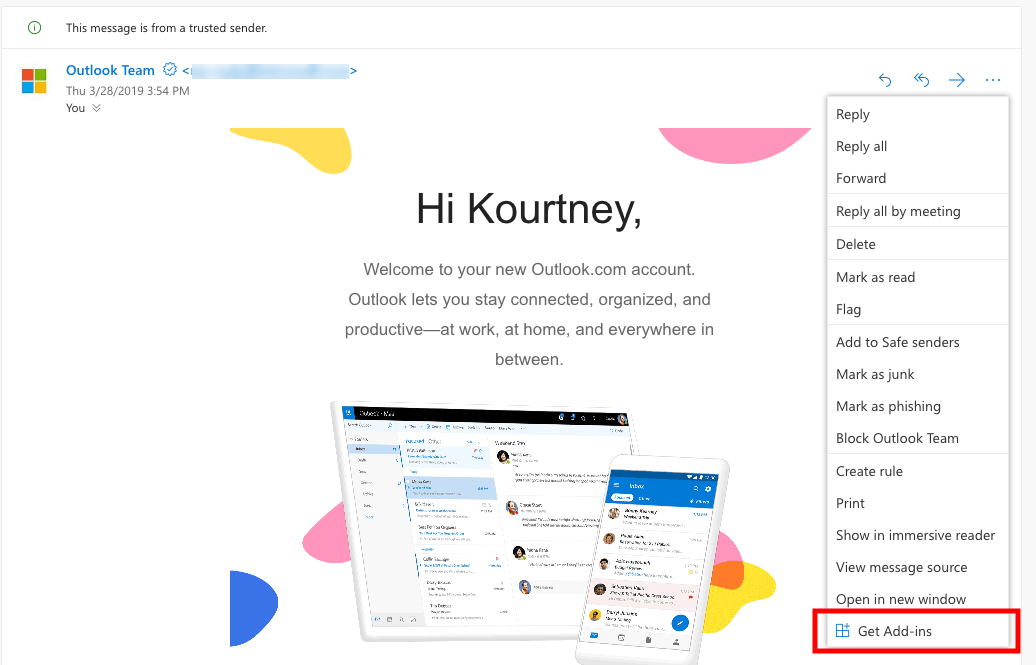The screenshot captures what appears to be an email from Microsoft, likely taken by someone setting up a new Outlook account. The interface is predominantly white. In the upper left-hand corner, there's a notification stating, "This message is from a trusted sender." Just below, the recognizable Microsoft logo—composed of four colored squares arranged into a larger square—is displayed alongside the sender's name, "Outlook Team," and their email address.

The email is dated "Thursday, March 28, 2019, at 3:54 PM." The subject of the email warmly welcomes the recipient, Courtney, to their new Outlook.com account. The body of the email highlights various features of Outlook, emphasizing its ability to keep users connected, organized, and productive whether at work, home, or anywhere in between.

Embedded within the email is an image displaying both a tablet and an iPhone, each showing the Microsoft Outlook application, symbolizing the app's compatibility across multiple devices.

Along the left side of the screen, numerous interactive options for handling the email are listed: Reply, Reply All, Forward, Reply All by Meeting, Delete, Mark as Read, Flag, Add to Safe Senders, Mark as Junk, Mark as Phishing, Block Outlook Team, Create Rule, Print, Show in Immersive Reader, View Message Source, Open in New Window, and Get Add-ins. Notably, the "Get Add-ins" option is emphasized with a red box drawn around it.